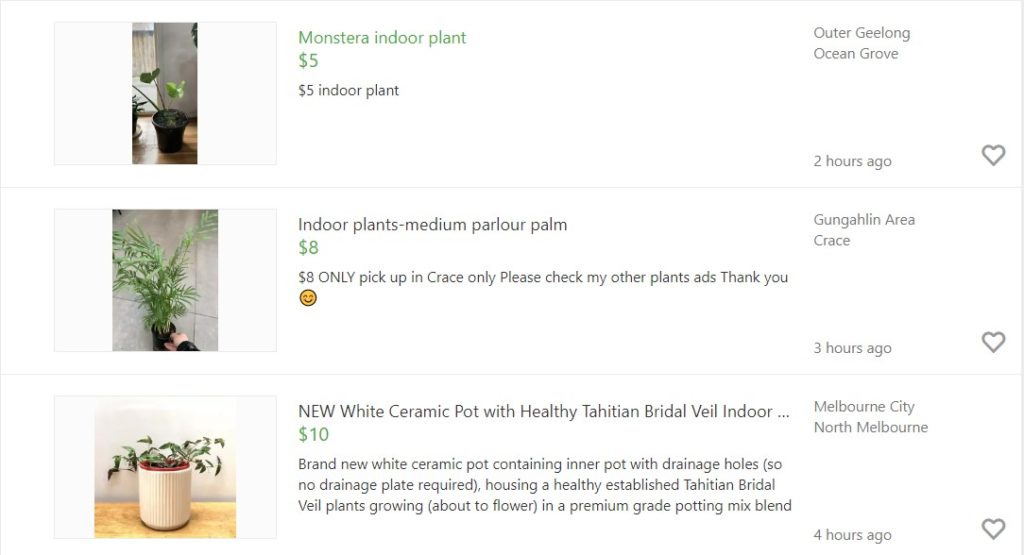The image is a screenshot of a plant-selling website, organized into three columns. The first column features images of the plants being sold, the second column contains detailed descriptions and prices, and the third column provides the location of the seller and the time since the post was made. Each listing also has a grey heart icon that users can click to "like" the post. 

At the top of the image, there's a listing for a Monstera indoor plant priced at $5. The description reads "Indoor plant, $5," and it’s located in Outer Geelong Ocean Grove, posted two hours ago.

The second listing shows an "Indoor Plants Medium Parlour Palm" priced at $8. The description states "$8, only pick up in Cres only. Please check my other plant ads, thank you." The location is listed as Gugahlin area, Cres, with the post made three hours ago.

The last listing features a plant in a white ceramic pot, though further details about this plant are not provided.